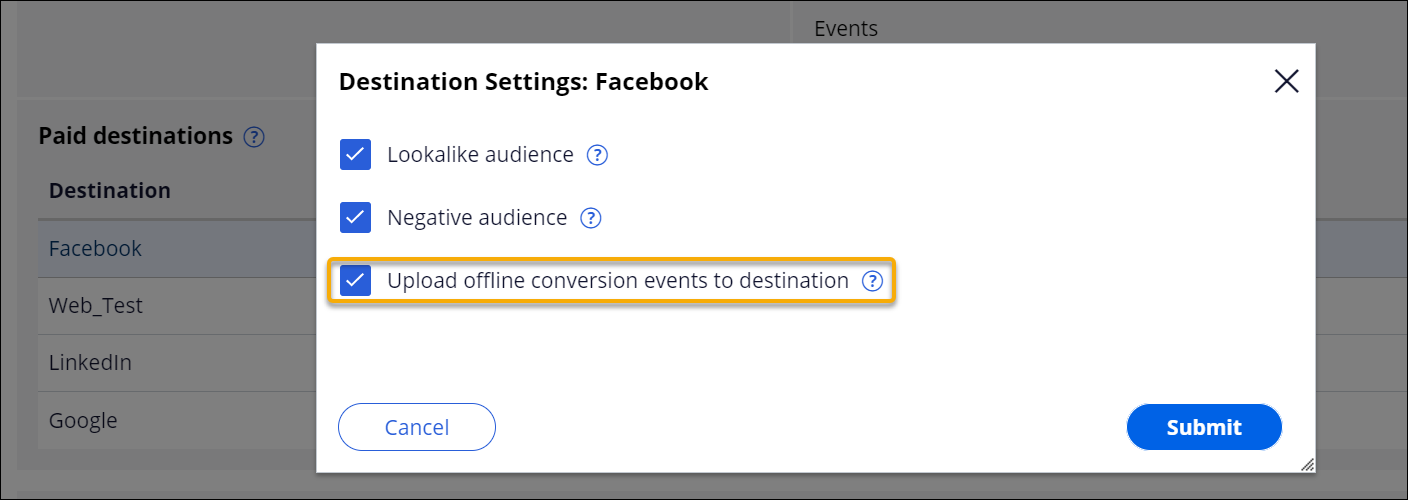The screenshot depicts a desktop interface, likely from a web application or browser-based software, given its wide aspect ratio. The user interface primarily features a lot of whitespace with black text. On the left sidebar, a vertical list of options is visible, including:

- Pay Destinations (with a question mark)
- Destination
- Facebook (highlighted in blue)
- Web_Test
- LinkedIn
- Google

The Facebook option is currently selected, as indicated by its blue highlight. A white pop-up menu titled "Destination Settings: Facebook" overlays the main content area. This pop-up includes a black 'X' button for closing the menu. 

In the pop-up, there are three items with associated blue checkmarks, each followed by a question mark icon for more information:

1. Look-Alike Audience
2. Negative Audience
3. Upload Offline Conversion Events to Destination (highlighted in orange)

At the bottom of the pop-up, there are two buttons: "Cancel" on the left in white, and "Submit" on the right in blue. 

The interface hints that the software might be related to web design or digital marketing, particularly focusing on audience management and conversion tracking. However, the exact purpose of the software is not immediately clear from the screenshot alone.